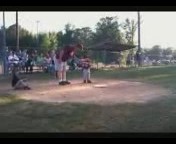This small, extremely blurry, and low-resolution thumbnail photograph depicts a baseball scene at a ballpark. The image captures a moment near home plate, where a central figure, a man possibly in khaki shorts or white shorts and a short-sleeved purple shirt with yellow numbers, leans over a young boy who is either his son or a player on the team. The boy is wearing a darker colored shirt, possibly purple with yellow numbers, and light blue or white pants, and appears to be holding or swinging a baseball bat. The field features a sandy, light brown circular patch at the center, indicative of the home plate area of a baseball diamond. In the background, there are some trees, light poles, and a line or stand of people who are likely watching the game, possibly seated on a bench or near a fence. Additionally, a black strip border runs along the top and bottom edges of the image. The sunlight shining on the field enhances the atmosphere of the scene.